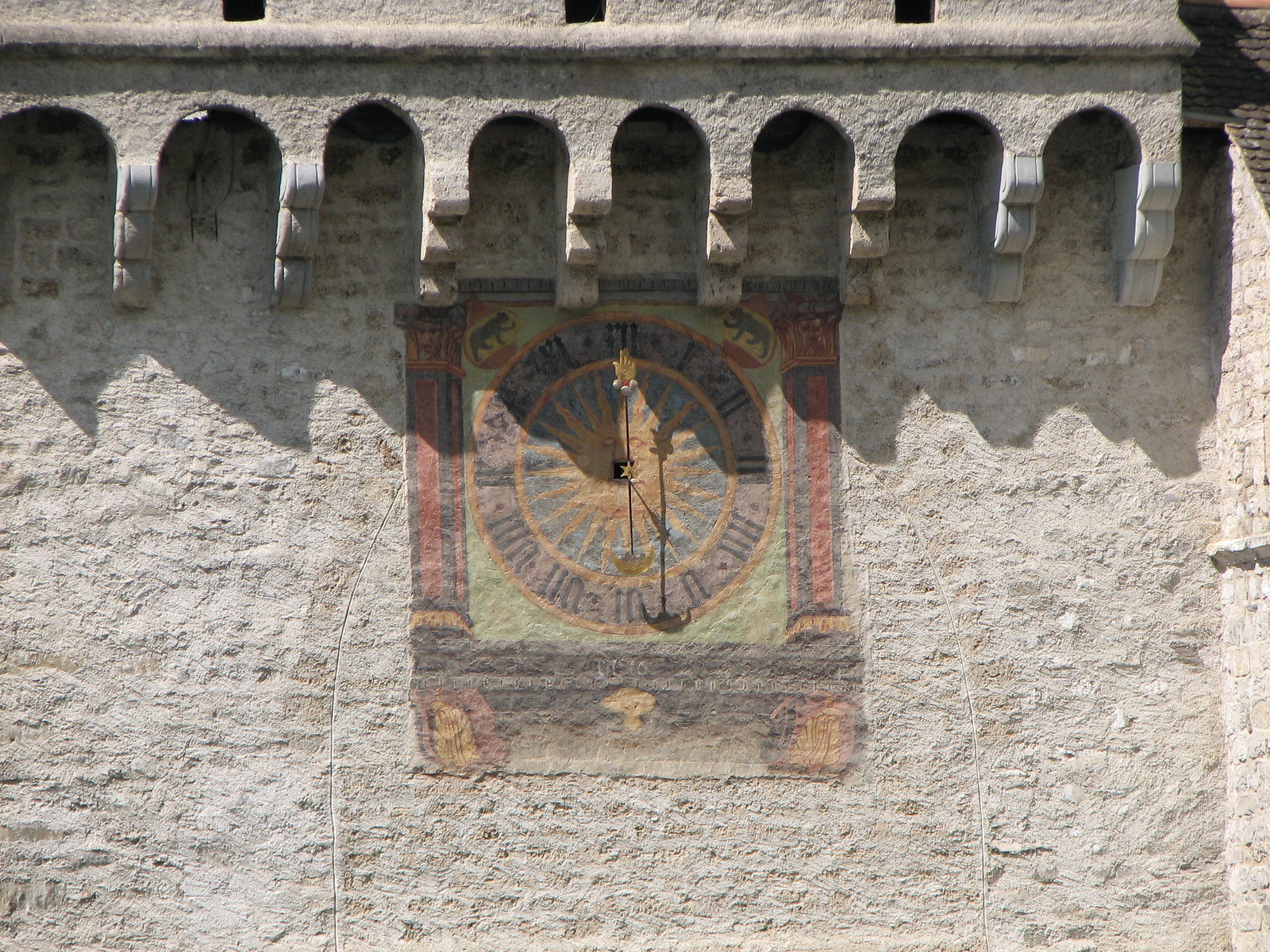This image showcases an antiquated and weathered stone building, characterized by its rough edges and aged facade. At the top of this old stone wall, there are small, rounded arches resembling windows, adding an additional layer of architectural interest. Below this, the wall features a striking, albeit faded, mural of a clock. This clock, painted directly onto the stone, presents a palette of red, black, and gold, with blue forming the clock's face. Distinctively, the clock’s center resembles a sunburst, and its Roman numerals are faint yet visible. The functioning clock hands extend outward, showcasing intricate designs with the minute hand shaped like an actual hand complete with a star at its base, and the hour hand resembling a lantern. The current time displayed by this unique clock is around six o'clock. Flanking the top corners of this painted clock are depictions of large felines, likely lions or cougars, adding a touch of majestic symbolism. Additionally, there are shadowy, black rectangles or yellow marks at the bottom corners of the clock face, hinting at further ornate designs or decorations. This combination of architectural features and the detailed, symbolic clock creates a captivating tableau of historical artistry.